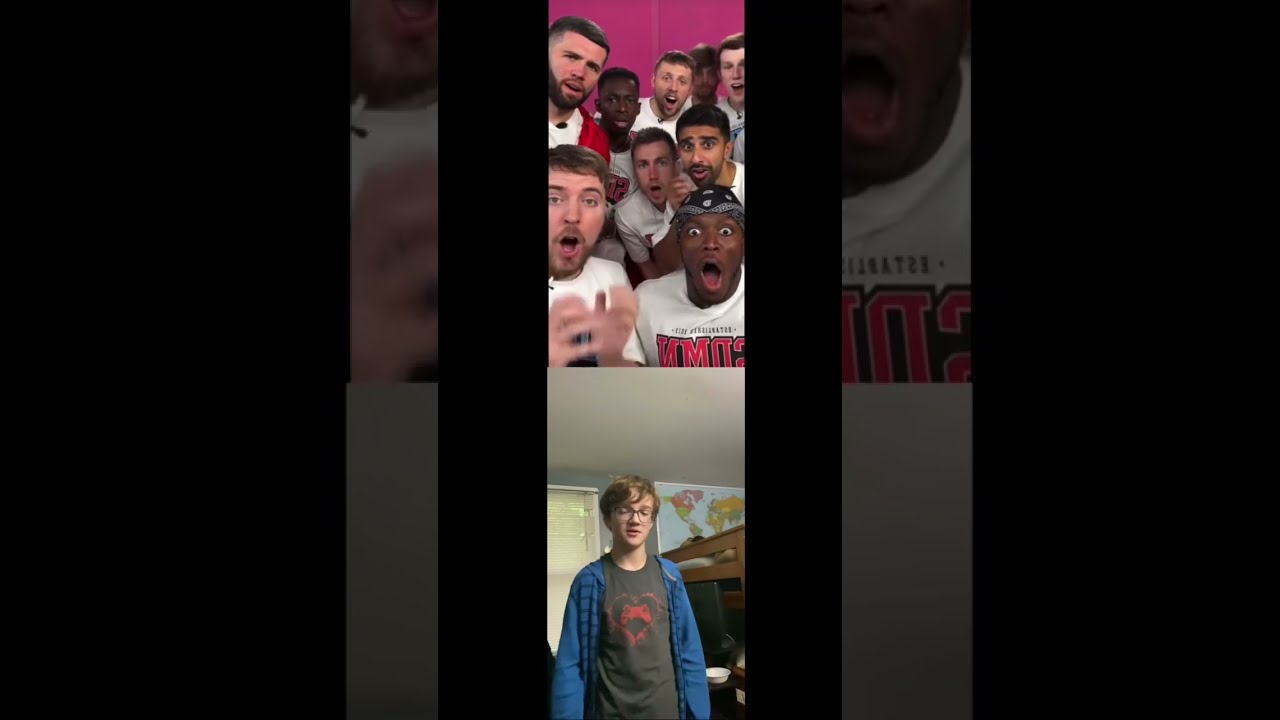The image captures a social media screenshot, possibly from TikTok or Instagram, featuring two vertically stacked photos encased in black borders. The top photo displays a diverse group of men, both white and black, wearing white T-shirts with the text "SDMN established" on them. They exude expressions of amazement, their mouths wide open in astonishment, and one man on the right sports a black bandana. Positioned against a red background, these men are reacting to something in the lower image. 

The bottom photo shows a young white boy with glasses and blonde hair, clad in a green T-shirt and a blue vest. He is standing in his bedroom, which contains a bunk bed, a world map poster on the wall, white window blinds, a black chair, and some furniture. The boy, looking down slightly, seems to be the focal point of the top image's reaction. The photo compositions and the stark contrasts between the two images suggest a reaction video format, capturing the intense surprise and curiosity of the reacting group toward the boy in his room.